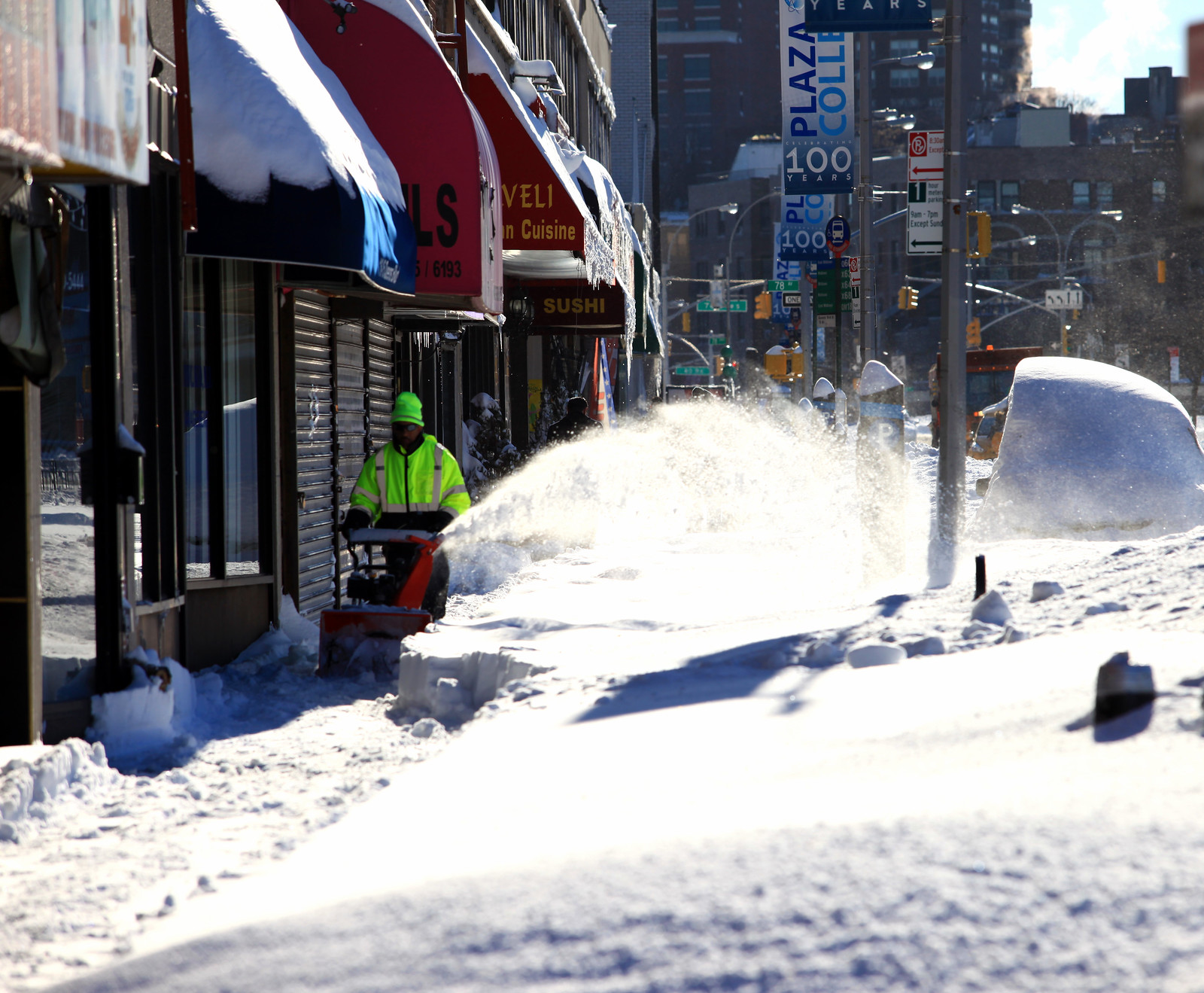This photograph captures a bustling city street, possibly resembling New York City, after a significant snowstorm. The sidewalks and streets are enveloped in up to two feet of snow, creating formidable barriers for pedestrians. A man with dark skin, attired in a high-visibility, electric-green reflective outfit and a fluorescent beanie, operates a red gas-powered snow blower. He works diligently to clear a path along the storefronts, which display a variety of colorful awnings—red, blue, and more. The snow, as it's expelled by the snow blower, forms towering piles along the edge of the sidewalk. Despite the heavy snow accumulation, the scene is brightly lit by the sun, suggesting a clear day that contrasts sharply with the wintry landscape. Further down the street, a yellow bus is visible, maneuvering through the barely cleared roads, adding a dynamic touch to this vivid portrayal of urban life post-blizzard.